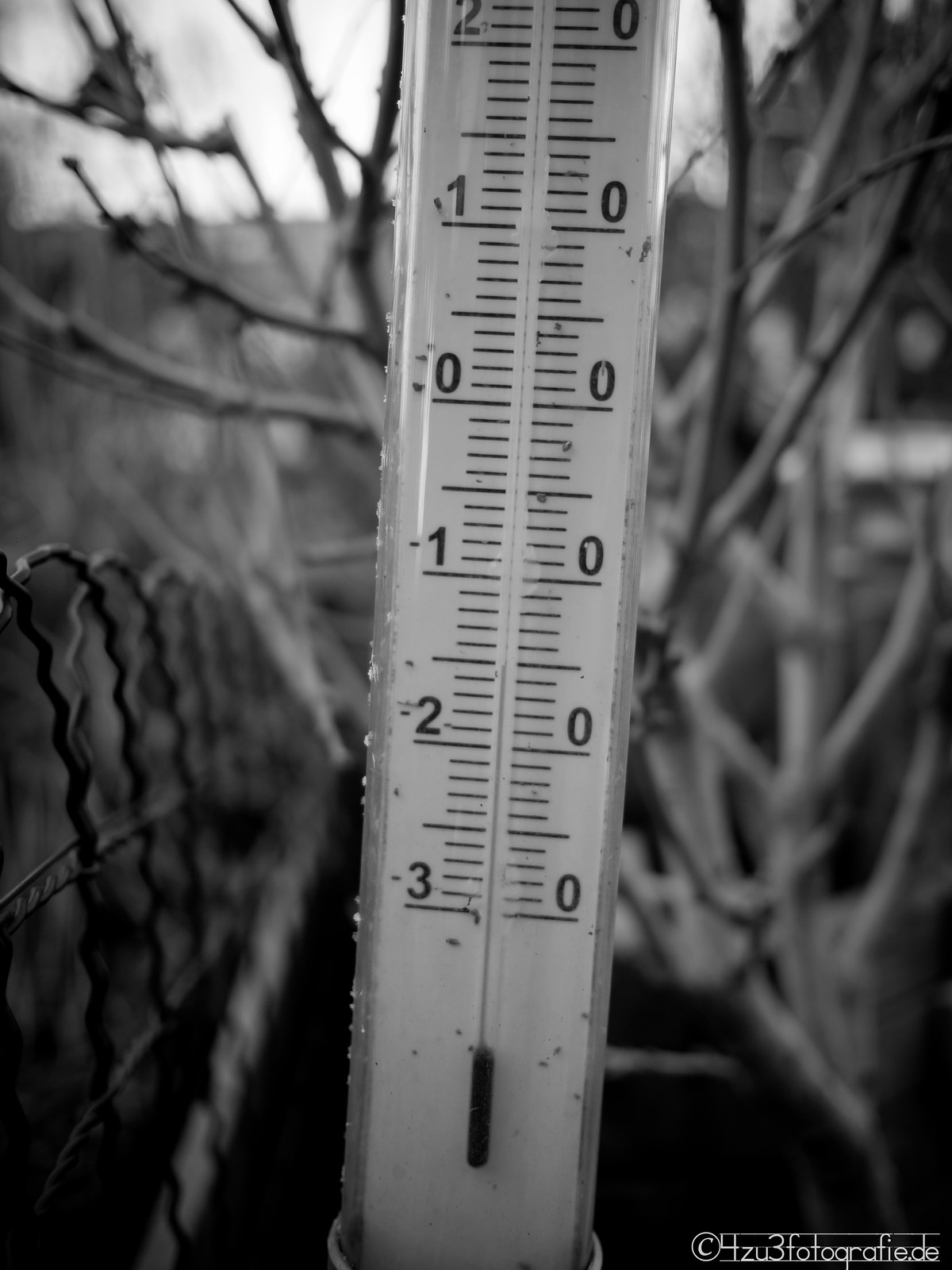A detailed black-and-white photograph features a close-up view of a thermometer. The bottom right corner includes a photo credit marked with a © symbol, followed by the text "4zu3fotografie.de" in a white typeface against a dark background. The thermometer's scale starts at negative three at the bottom and ascends through negative two, negative one, zero, and positive numbers up to two. Notably, there are four hash marks between each major numerical increment, including a halfway mark, meticulously representing the temperature gradations. The thermometer's mercury or indicating fluid is situated well below the negative three mark, suggesting extremely cold temperatures. The background subtly reveals out-of-focus branches devoid of leaves, likely accompanied by a garden fence, enhancing the wintry, barren ambiance of the scene.